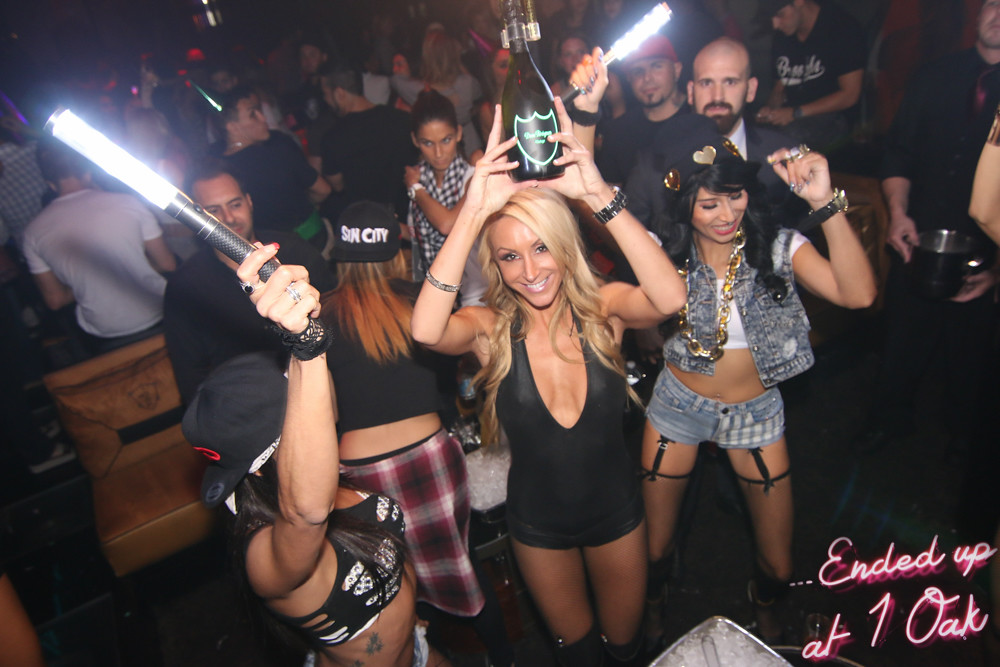In this energetic image from a nightclub party, a blonde woman stands at the center, exuding confidence in a tiny, skin-tight black mini dress while holding a dark bottle of champagne or wine with a green label high above her head. She has a strikingly tanned complexion and slim figure. Flanking her on either side are two women: to the left, a Latino woman sways in time with the music, sporting very short shorts, a big gold chain, and a backwards hat while gripping a mini light stick resembling a lightsaber. To the right, another woman, tanned with a hat and a revealing crop top, dances energetically, wearing short denim shorts and stockings, also holding a light stick. The background bustles with a dimly lit crowd, blurred but visibly engaged in their euphoric activities of dancing, drinking, and mingling. At the bottom right corner, the words "ended up at 1 OAK" subtly overlay the scene, grounding the vibrant image in a renowned nightlife destination.